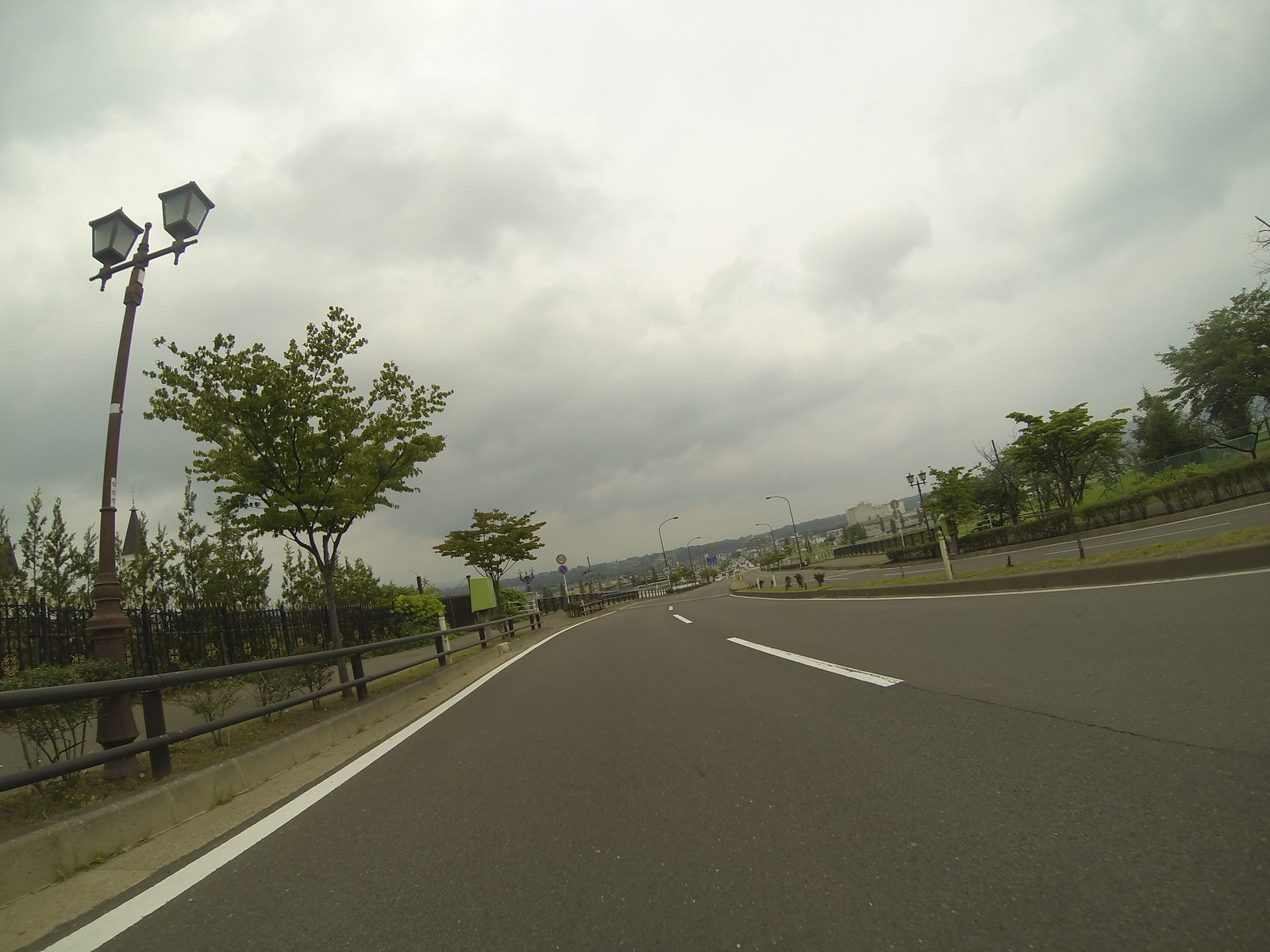In this outdoor image, we see a curved highway with two lanes in each direction, separated by a green grassy median. The black asphalt road features white lines, and there are no visible cars in the immediate vicinity, though some might be farther back. Under a heavily overcast sky filled with gray and white clouds, the scene looks as though it could rain soon.

On the left side of the road stands a large brown metal lamppost with two old-fashioned lights, which are currently off. Alongside it, there is a wrought iron fence, and further back on the sidewalk, we see standard streetlights typically found above highways. Lush green trees filled with leaves line both sides of the road, adding a touch of nature to the scene. In the distance, the view narrows, showcasing more of the road and additional trees. A faint silhouette of a gentleman can be spotted on the sidewalk down the road, adding a human element to the expansive and detailed landscape.